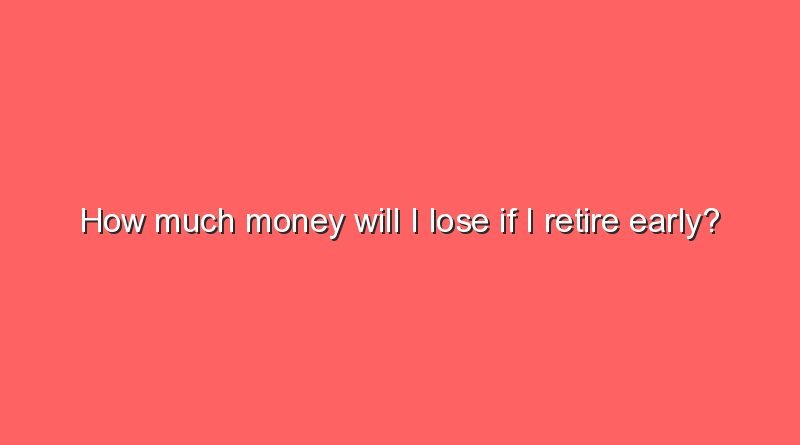The image features a horizontally long rectangular background, predominantly in a salmon pink color. Centered on this backdrop is a concise question rendered in thin white text with a subtle black shadow for emphasis, reading, "How much money will I lose if I retire early?" The sentence, notable for its small font size, is the only content on the image and leaves substantial empty space around it. The text is entirely in lowercase except for the initial "H" in "How," adding a slight informal touch to the presentation. The overall layout and design are reminiscent of a minimalist PowerPoint slide.